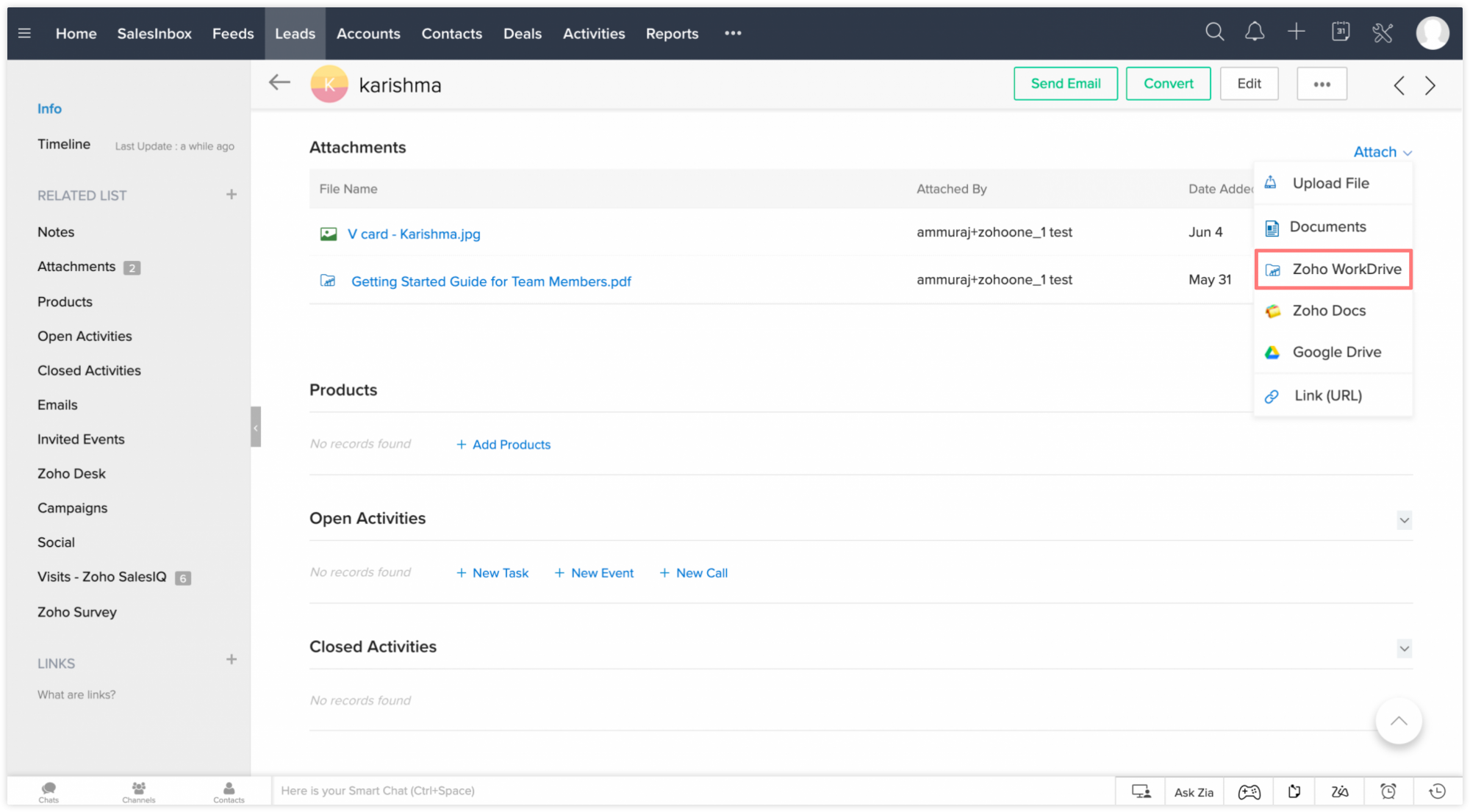This is a screenshot of a business-oriented web page. The page features a clean white design with a user interface designed for easy navigation and functionality.

- **Top Bar:**
  - The top bar is a dark charcoal gray, contrasting sharply with the rest of the page.
  - On the far left, there is a white hamburger menu icon (three horizontal lines), followed by a white text-based navigation menu with the following options: Home, Sales, Inbox, Feeds, Leads, Accounts, Contacts, Deals, Activities, Reports.
  - Three ellipsis dots hint at additional menu options available in a drop-down.
  - On the far right, there is a series of icons: a white magnifying glass for search, a notification bell, a plus sign (likely for adding new items), a square icon (unclear in function), an icon combining a wrench and screwdriver for settings, and a profile icon depicting a white silhouette of a person on a light gray background.

- **Left Menu:**
  - This section has a light brown background and includes various navigation options with bold text for emphasis.
  - Options listed in this menu include Timeline, Notes, Attachments, Products, Open Activities, Closed Activities, Emails, Invited Events, Zoho Desk, Campaigns, Social, Visits, Zoho Sales, and Zoho Survey.

- **Main Content Area:**
  - Mostly white with blue hyperlinks and occasional bolded text for important sections.

- **Attachment Menu (Right Section):**
  - Under a drop-down labeled "Attach," there are several options highlighted with a red border: Upload File, Documents, Zoho Work Drive, Zoho Docs, Google Drive, and Link URL.

This page seems to be a part of a Zoho business application suite, facilitating comprehensive management with its various tools and integrations.